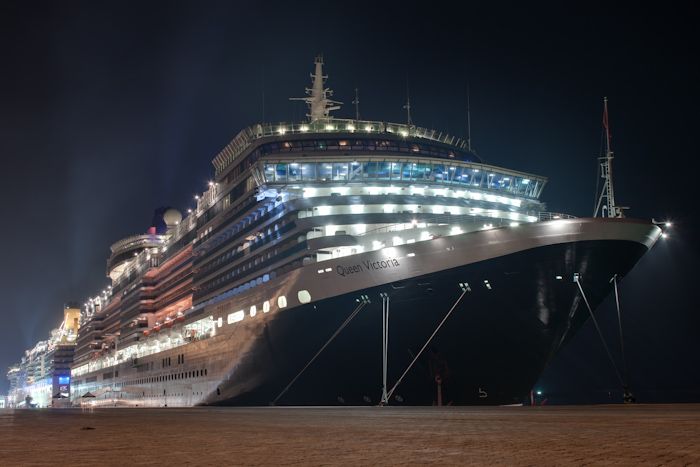The image depicts a nighttime photograph of the impressive cruise ship, Queen Victoria, docked beside a large, empty, brown stone platform. The ship, illuminated by a combination of white, blue, orange, and yellow lights, creates a striking contrast against the dark sky. The vessel's name, "Queen Victoria," prominently displayed in dark letters on its black hull, signifies its grandeur. The photograph captures a clear view of the ship's front and side, revealing multiple stories—five above the deck and an estimated four to five below—emphasizing its immense size and luxury. Smokestacks rise from the rear, while the antenna is visible towards the front. The ship is anchored to the dock with visible ropes, but no people or other identifying details are present in the image. There's an ambiguity about whether the ship extends far into the distance or if there is another ship nearby, contributing to the sense of its vast length.